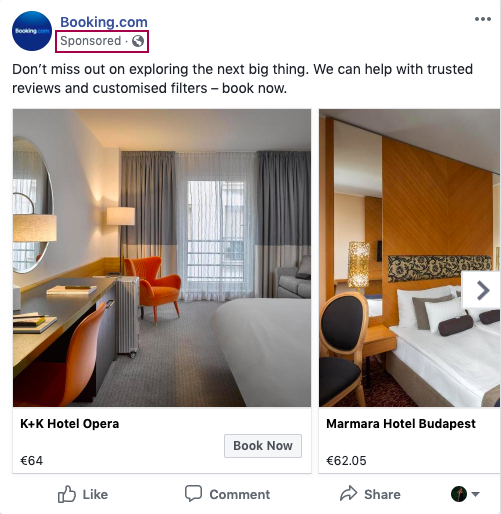This image is a screenshot from Booking.com. In the top left-hand corner, there is a blue circle with "Booking.com" inside it, followed by "Booking.com" in blue text. Below that, within a pink rectangle, it says "Sponsored."

On the white background, black text reads: "Don't miss out on exploring the next big thing. We can help with trusted reviews and customized filters. Book now."

Displayed below the text are two images of different hotel rooms. The larger image on the left showcases a room from K&K Hotel Opera, priced at 64 euros. This room features a white-covered bed positioned at the bottom right-hand corner. The backdrop of the image highlights large windows adorned with gray and light gray curtains. An orange armchair and a gray couch add contrasting hues to the room's decor. Along the left side of the photo, two lamps are visible: a tall standing lamp behind the orange armchair and a desk lamp. A round mirror adorns the wall above a wooden desk, complemented by an orange desk chair pushed in neatly.

To the right is a smaller image of a room at Marmara Hotel Budapest, priced at 62.05 euros. Dominating the room is a large bed with a white cover and dark gray pillows, set against a wooden wall with large mirrors. A glittery bedside lamp enhances the room's ambiance, while a wood and dark gray chair sits at the bottom left-hand corner.

Both images offer options to book now, like, comment, or share the listings.